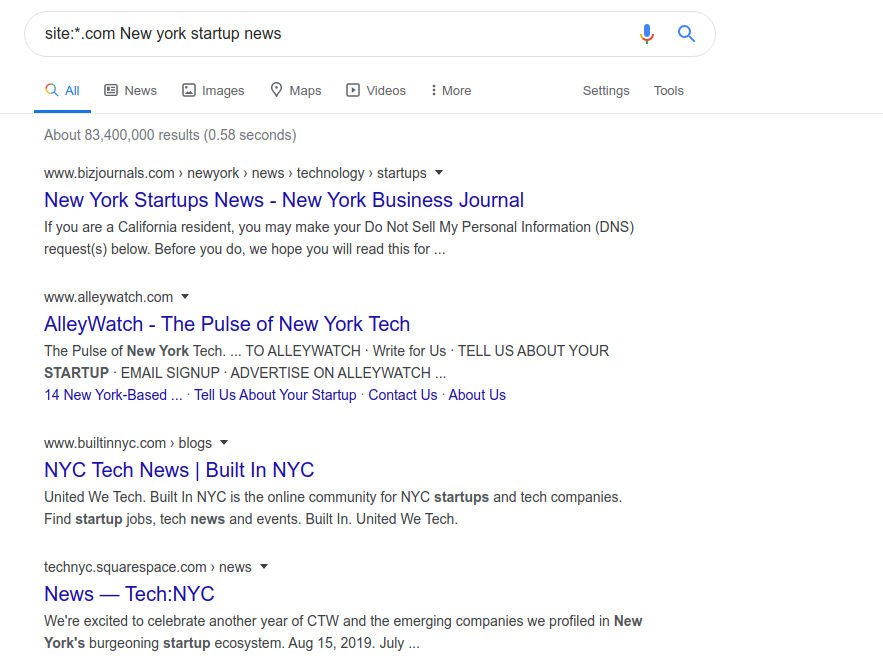The image displays a search engine results page (SERP) with various sections and tools. At the top, there is a gray-outlined rectangular search bar that bulges into circular shapes on either end. Within the search bar, there are icons: a microphone on the left and a magnifying glass on the right. Below this, the search options are laid out with colorful icons. 

- "All" is displayed in blue text with a blue underline, followed by a black outlined square with dashes containing the word "News."
- A black outlined square with an image icon labeled "Images," 
- Followed by a map symbol labeled "Maps."
- Another gray outline square with an arrow pointing right labeled "Videos."
- Three dots representing more options.
- To the right, there are links labeled "Settings" and "Tools."

The search results are listed beneath these options. The first result in gray text with some darker gray text next to an arrow pointing down reads, "New York Startup News - New York Business Journal." Below this is the result description in black text followed by the website URL with an arrow pointing down.

The second result has "Alley Watch - The Pulse of New York Tech" in blue text followed by additional information in black text, then the website URL with an arrow pointing down.

The third result reads, "NYC Tech News - Built In NYC" in blue text followed by a description in black text, then the website URL with an arrow pointing down. 

Finally, the fourth result is labeled "News - Tech: NYC" in blue text, followed by a description in black text.